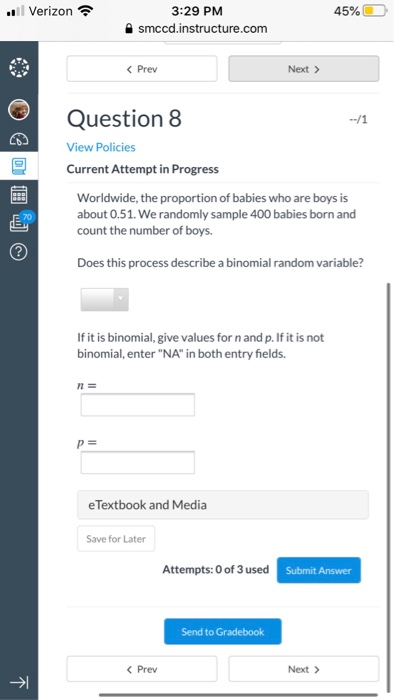The image depicts a mobile device screen capture of a web page with a clean, white background. At the top of the screen, there are two navigational buttons: the one on the left, which blends into the white background, features a left-pointing arrow indicating "previous"; the button on the right is a light shade of grey and has the word "Next" accompanied by a right-pointing arrow. 

Centered prominently on the page is a large, bold black text indicating "Question 8". Just below this, a clickable blue text link reads "View Policies". Following this, the text "Current attempts in progress" is displayed in regular black font. Under this section, additional explanatory text is visible in black.

Towards the bottom of the page, the layout includes two empty text boxes. The first text box is labeled with "N =" directly above it, while the second text box is similarly labeled with "P =". This setup provides clear areas for user input in response to the question.